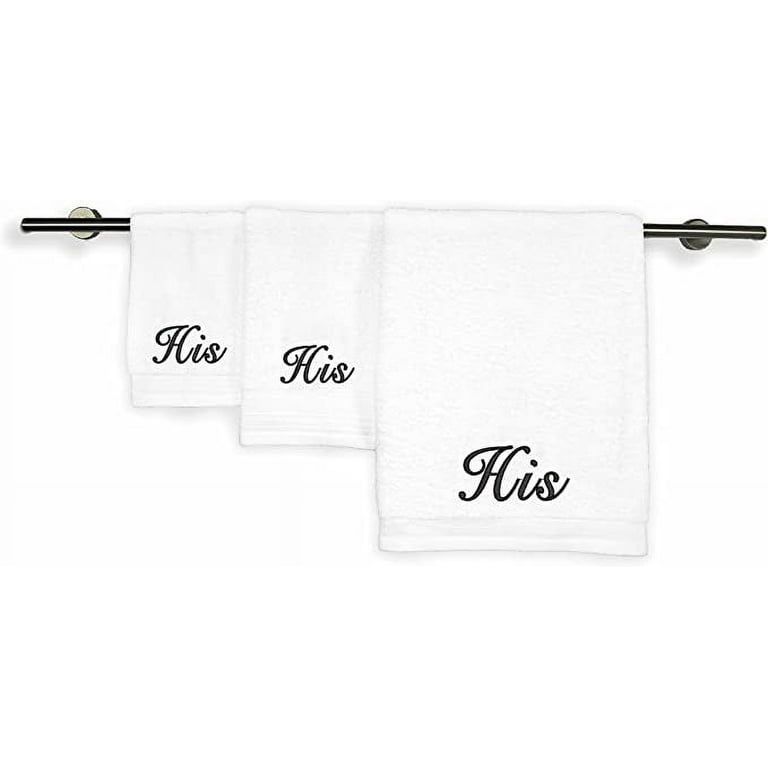The image showcases a minimalist and potentially product-oriented advertisement featuring three white hand towels of varying sizes—small, medium, and large—from left to right. Each towel is embroidered with the word "HIS" in an elegant cursive black font, centered about two inches from the bottom. They are neatly arranged on a slim, glossy black towel bar, which is affixed to a plain white backdrop. The backdrop creates an illusion of depth, making it difficult to discern the actual setting, though it is assumed to be a bathroom. The towels display a subtle decorative element, characterized by a slightly depressed border on the right and bottom edges, adding a touch of sophistication. Additionally, the towel bar is supported by two round brackets that add both support and a sleek, modern aesthetic.